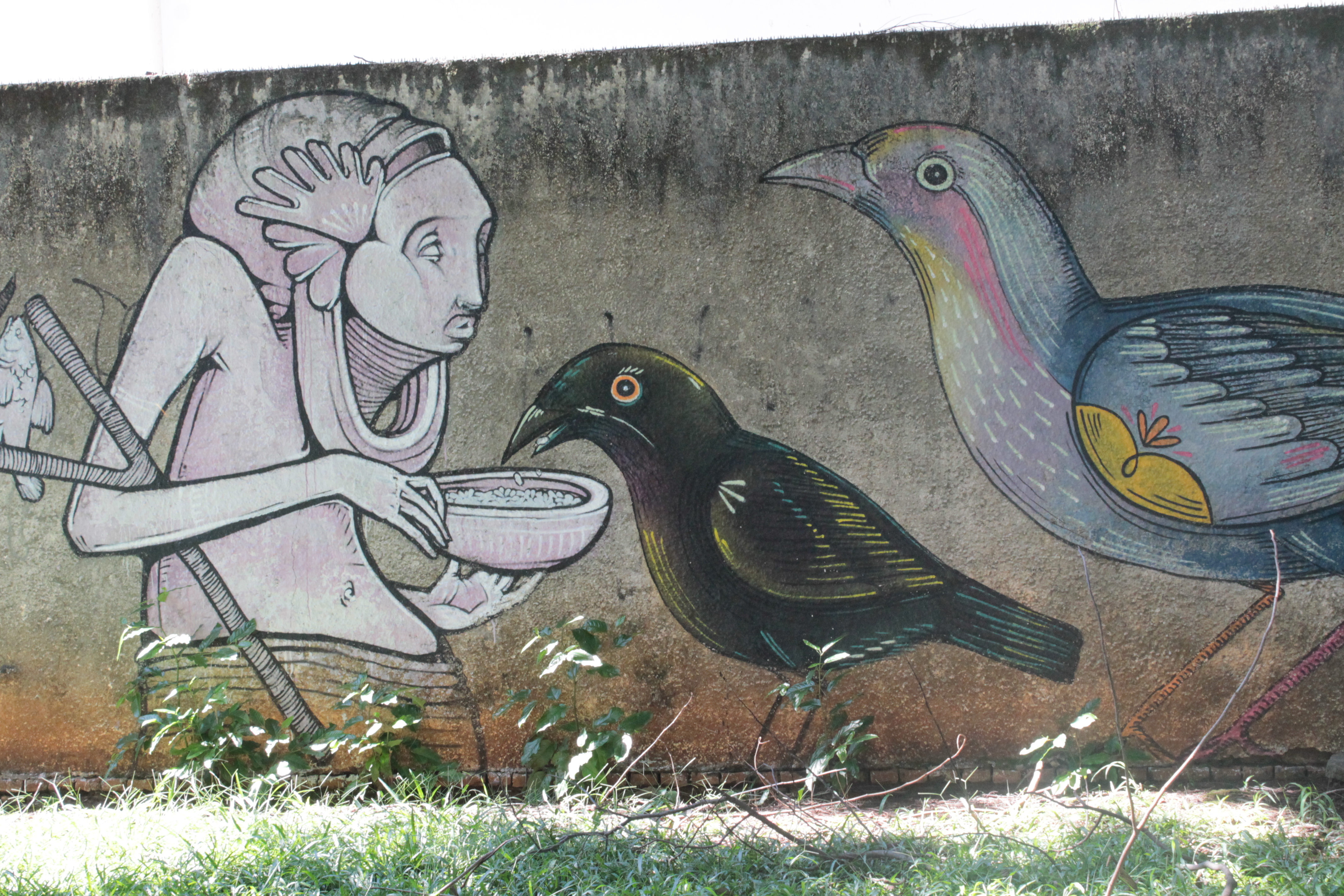The image showcases a detailed mural painted on a beige-gray concrete wall. The mural captures a vibrant scene with a shirtless man wearing a loincloth and a headdress extending under his chin. He’s holding a bowl filled with seeds, and a slender Y-shaped stick rests in the crook of his elbow, appearing to hold a fish. A prominent black bird, highlighted with yellow and blue accents, is perched on the bowl, feeding from it. Behind this bird, a larger avian figure, resplendent in hues of red, blue, yellow, pink, and white, waits its turn to feed. In the foreground, the mural is framed by real-life grass and trees, with branches adding an element of depth to the scene.